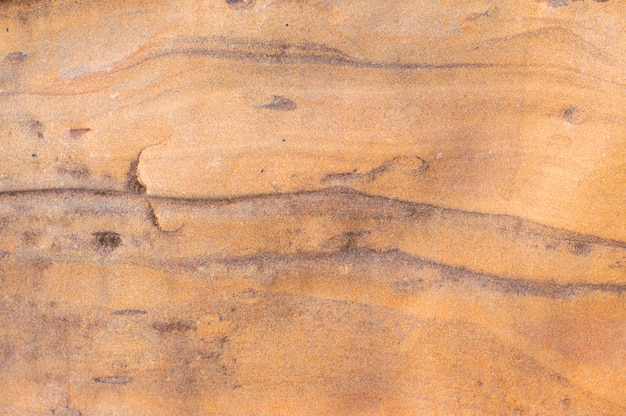The image presents a detailed and marbled surface, evoking the appearance of either a painting or a richly textured photograph. Dominating the scene is a fusion of burnt orange and off-white hues, swirled together to create a vibrant marbled effect. The top of the image showcases mostly these orange and white colors, with a subtle, faded black line interspersed with sporadic black spots and swirls. In the center, a thicker, prominent band of dark, almost black color runs horizontally across the image, breaking up the orange and white patterns. This central dark band appears to transition into a mixture of orange and mocha colors towards the bottom, with additional dark specks and swirls subtly decorating the surface. The texture of the material features lines, spots, and grooves, deepening the sense of intricacy. The marbling effect and the variation in colors suggest a natural beauty, reminiscent of a cave wall's surface or the weathered, detailed grain of a piece of wood. The overall composition, with its cracking lines and dark streaks, lends the image an organic, almost ancient feel, as though it belongs in an art museum or is part of a naturally occurring geological formation.